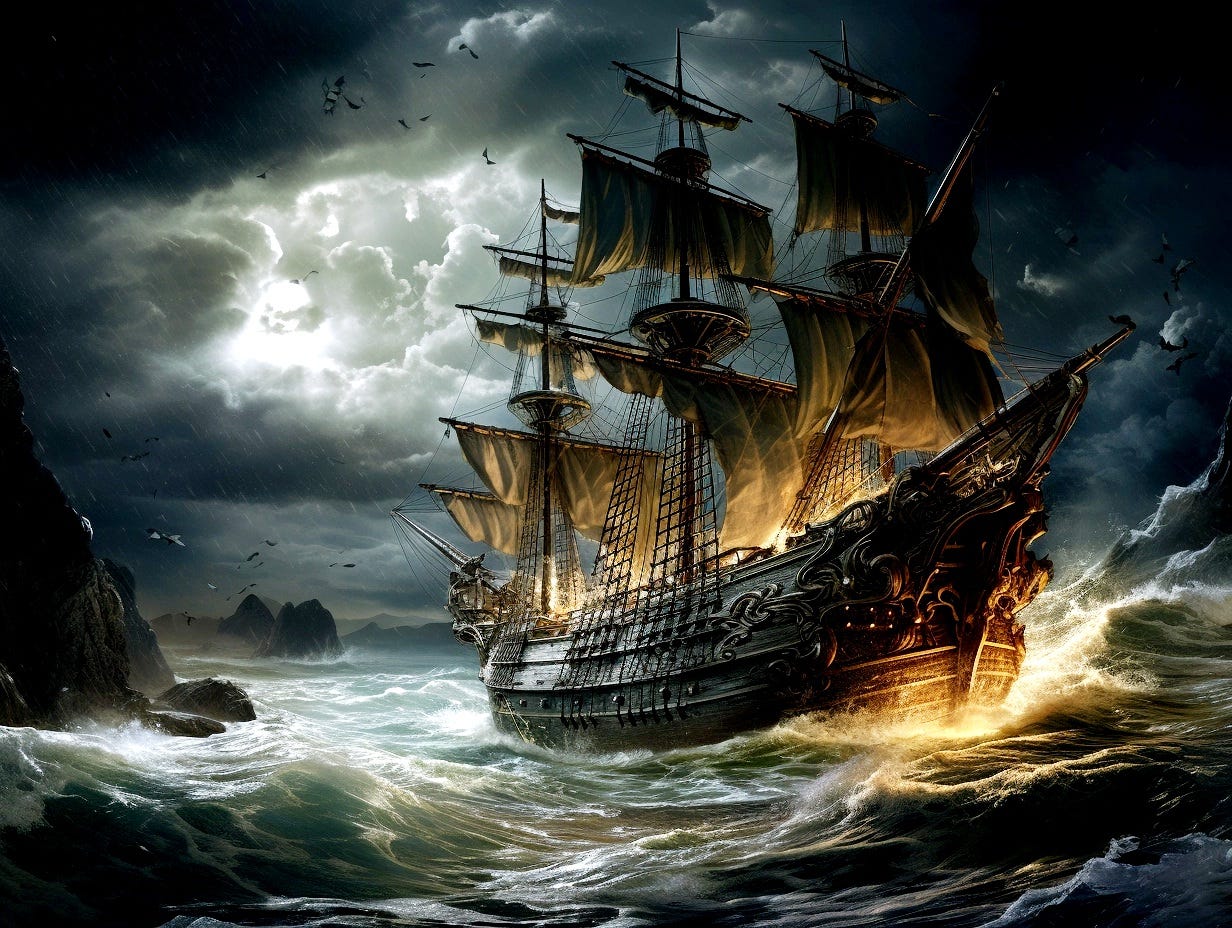This image depicts a detailed and intricate computer-generated or artistically drawn representation of a classic pirate ship navigating through a violent storm at night. The rectangular image primarily focuses on the dark and stormy atmosphere, with thick, ominous dark blue clouds blanketing the sky. There is a single break in the clouds just to the left of the center, allowing a beam of light—possibly moonlight or sunlight—to pierce through, illuminating part of the tumultuous scene below.

The ocean below the ship is extremely tumultuous, with massive, violently crashing waves adorned with white caps and foam. The water, tinted with a greenish hue, is interspersed with jagged brown rocks that jut menacingly from the surface, creating hazardous conditions for navigation.

The pirate ship itself is a marvel of design, a brown wooden vessel featuring elaborate and ornate inlays along its sides and front. It has a classic clipper ship form, with pointed ends and three to four towering masts, each adorned with large, billowing yellow sails. Nets are draped over the sides of the masts, ascending in a triangular shape towards the crow's nests atop the masts. The entire scene is dynamic and intense, capturing the perilous and adventurous spirit of a pirate ship caught in the throes of a dark stormy night. Birds can be seen flitting through the chaotic skies, adding to the dramatic and high-seas atmosphere of the artwork.